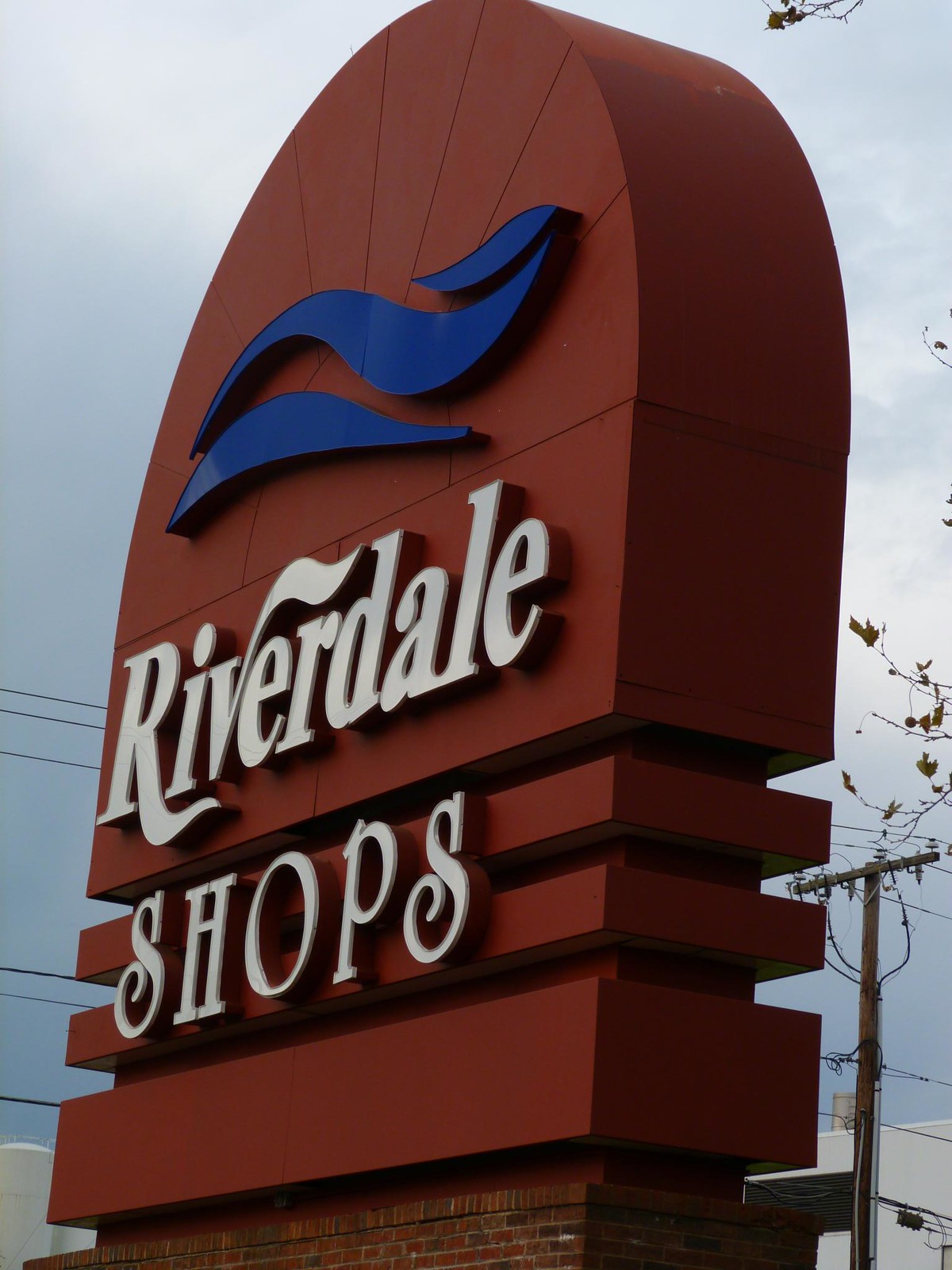The photograph captures an outdoor scene with a large, maroon sign angled to the left, prominently displaying the words "Riverdale Shops" in bold white, raised letters. The sign, which serves as an advertisement for a shopping center, is rounded at the top and features a striking blue wave graphic, symbolizing water, just above the text. In the background, a cloudy sky forms a dramatic backdrop, while power lines run horizontally across the lower half of the frame. A power pole is partially visible in the bottom right corner, and small branches and leaves intrude from the right-hand side, adding a touch of natural greenery to the otherwise industrial setting.